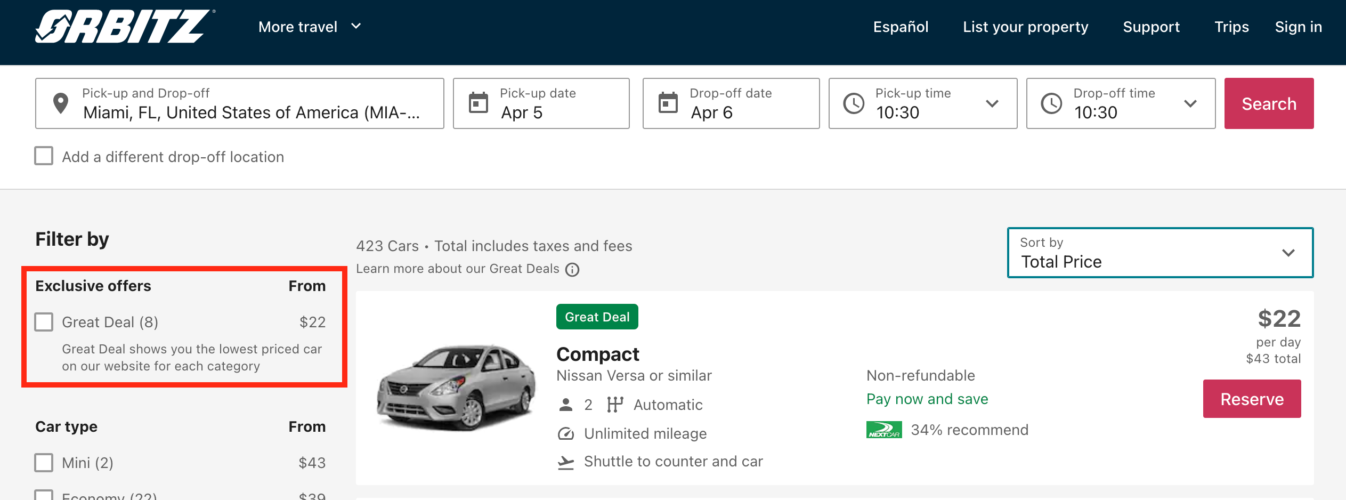Here is a cleaned-up and detailed caption for the image:

---

This image showcases the Orbitz website interface for car rental bookings. The top left corner prominently displays the "Orbitz" logo. Across the top of the page, set against a black background, there are several navigation options: "More Travel," "Español," "List Your Property," "Support," "Trips," and "Sign In."

Below this menu, a form is visible for selecting car rental details. The form fields include "Pick-up Location" and "Drop-off Location," with "Miami, Florida, United States" specified for both. The "Pick-up Date" is set to April 5, and the "Drop-off Date" is April 6. The "Pick-up Time" is listed as 10:30 AM. An option to "Add a Different Drop-off Location" is also available.

The search results indicate "423 cars" available, with a note that the "Total includes taxes and fees." There's an informational link encouraging users to "Learn more about our great deals." A sorting feature is present, labeled "Sort by Total Price."

One highlighted car option features an image of a gray sedan. Next to it, inside a green box, is the tag "Great Deal, Compact, Nissan Versa or similar." Additional details include an icon of a person with the following attributes: "Automatic," "Unlimited Mileage," "Shuttle to Counter and Car," "Non-Refundable," and "Pay Now and Save," along with a recommendation percentage of "34% Recommend." The price for this option is shown as "$22 per day, $43 total," and a red "Reserve" button is present for booking.

On the left-hand column, there's a "Filter By" section, followed by a red-bordered box labeled "Exclusive Offers." Inside the box, it reads "From $22," and mentions "Great Deals," indicating that 8 options are available in this price range. A note clarifies that "Great Deals show you the lowest priced car on our website for each category."